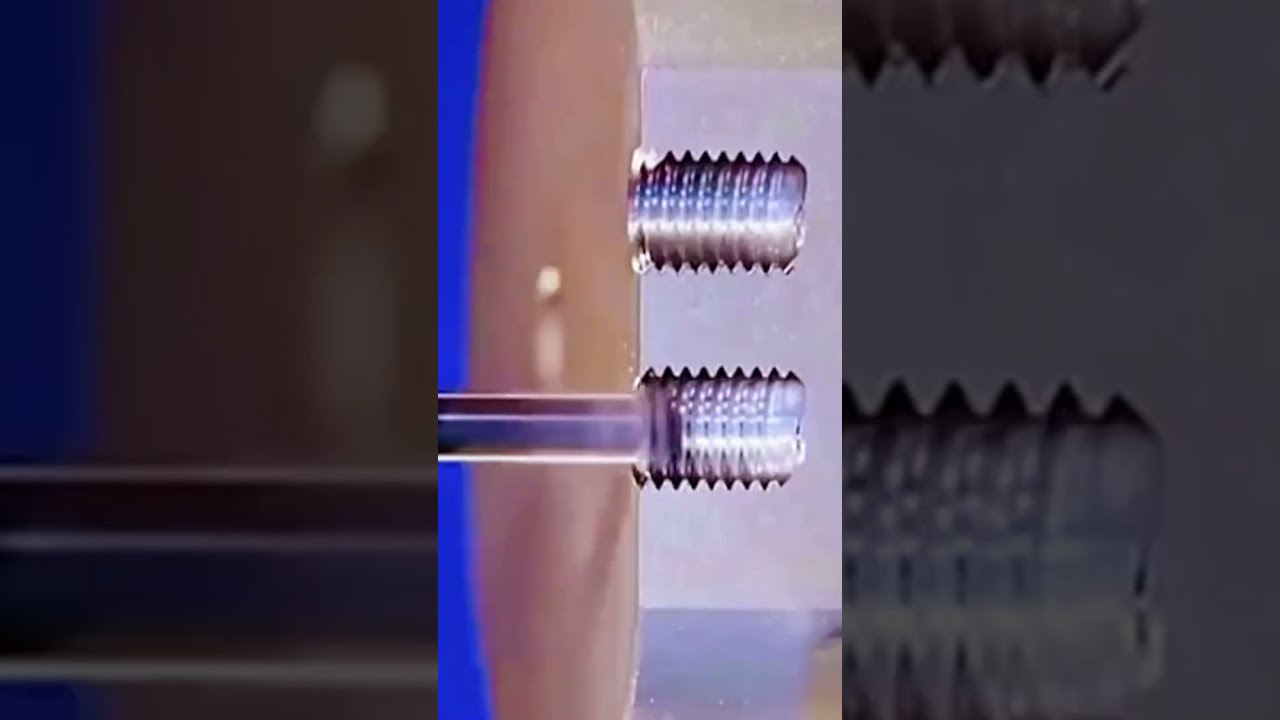This close-up image shows two metallic, screw-thread bolts placed horizontally and abutted against a light pink, vertically oriented object. Each bolt, featuring about eight distinct threads, emerges from a brownish surface and extends to the right side of the image. One of these bolts is connected to a clear tube. A blue vertical line and a white background provide a stark contrast to the machinery. The image, framed vertically, includes mirrored close-ups of the central section on both the left and right sides, adding a layered visual effect. The background appears slightly pixelated and blurry, with shades of gray and a prominent blue streak running from the bottom left to the top left, suggesting it may have been taken from a camera phone.